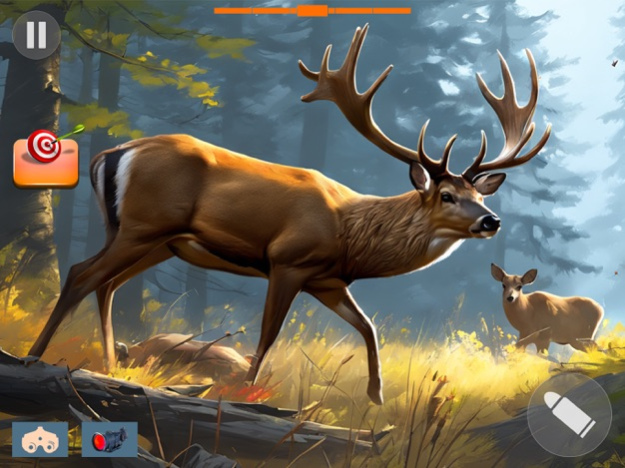This detailed screenshot from a video game depicts a cartoonish outdoor, nature-themed setting, resembling a large forest with numerous trees, grass, logs, and rocks. Dominating the foreground is a muscular, large buck with prominent antlers, a brown coat, black eyes, and a black nose. Adjacent to it on the left is another deer, partially concealed in tall grass, appearing to be shot. To the right background, a smaller deer without antlers gazes toward the viewer. 

The game interface presents various elements: an orange progress bar at the top, a pause button on the left, and a bullseye target with an arrow below it. Further down on the left are two icons resembling different types of scopes—one white with the number three, and another with a red center. On the bottom right is a gray circle featuring a white bullet icon.